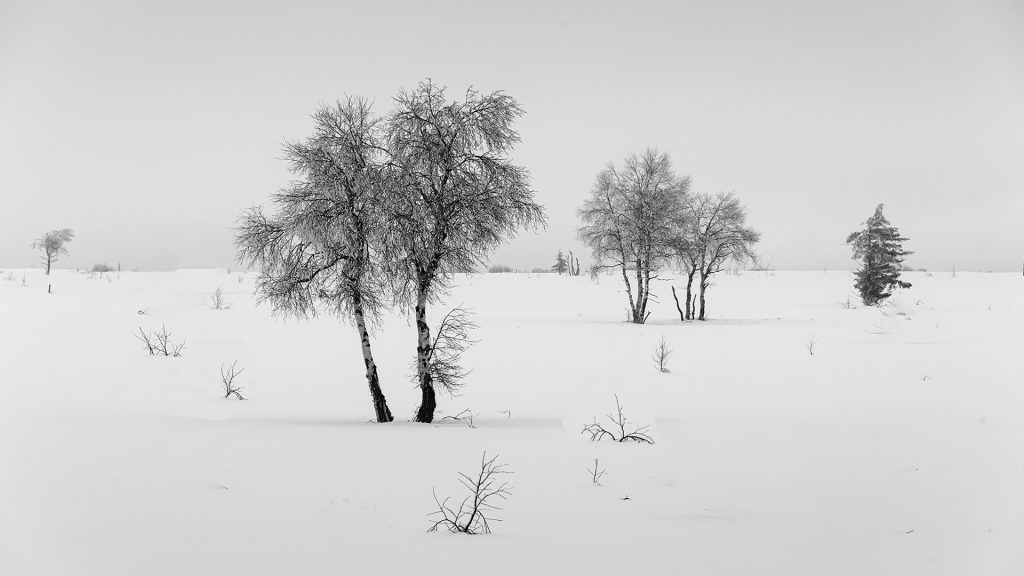The image presents a serene winter landscape blanketed in snow, captured in black and white. The sky is a grayish white, blending subtly into the completely snow-covered ground. Near the middle of the scene stand two tall trees, their branches laden with snow. To the right of these, slightly further back, are three more snow-covered trees, and to their right stands another solitary tree. Scattered throughout the snowy expanse are tiny branches protruding from the ground, hinting at smaller, buried shrubs. The stark landscape, devoid of typical forest foliage, highlights about eight trees, their silhouettes stark against the monochromatic backdrop of the sky and land. The overall scene evokes a calm, open space overwhelmed by winter's embrace, with the gray tones of the sky only slightly distinguishable from the white of the snow.